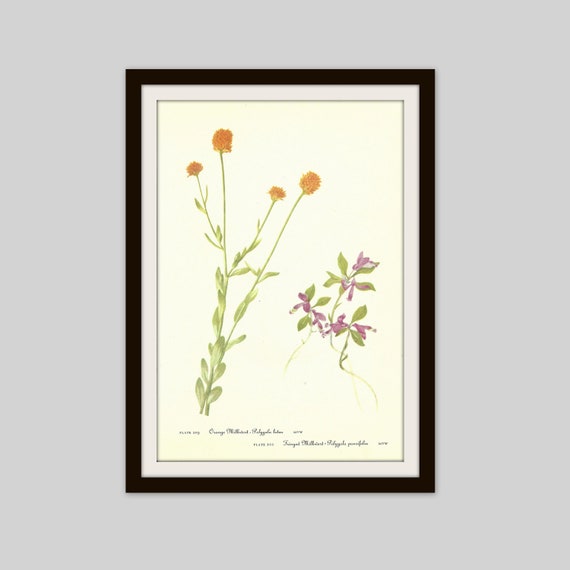The image depicts a framed botanical illustration against a pale gray, silvery wall. The frame is simple and black, with a white matting that provides a clean border around the artwork. The illustration itself is on ivory-colored paper and showcases two different flowering plants arranged side by side. 

On the left, there is a yellow-flowered plant with small, clover-shaped blossoms clustered tightly together. This plant has clasping small green leaves that cling to its stem. On the right, there is a smaller plant adorned with tubular-shaped purple flowers and a few clover-shaped leaves. Below each plant, there is cursive writing that includes the scientific and common names of the plants, as well as the dates, though these details are too small to be clearly discerned from the photograph. The overall presentation of the illustration exudes an old-fashioned botanical style.